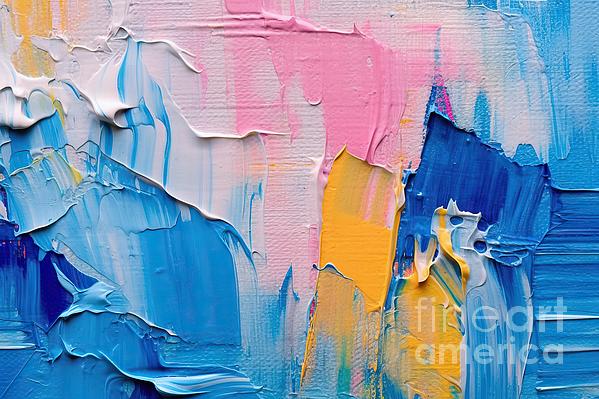The image resembles an abstract painting with a highly textured surface, almost as if cake frosting has been spread across a canvas. The left side features shades of dark blue, light blue, sky blue, and white, with a touch of yellow at the top. As you move toward the middle, the colors transition into light pink and a darker, Pepto-Bismol pink. The bottom section is a bright yellow, and the right side reintroduces dark and light shades of blue interspersed with white at the top. The overall composition looks smudged and layered, with the paint appearing thick and creamy, as if it might drip. A watermark reading "Fine Art America" is visible in the lower right corner. The painting's colors and textures are illuminated from above, suggesting display lighting, possibly in an art museum. While the paint looks wet, it is likely dry, adding to the illusion of dripping, richly applied frosting-like strokes.